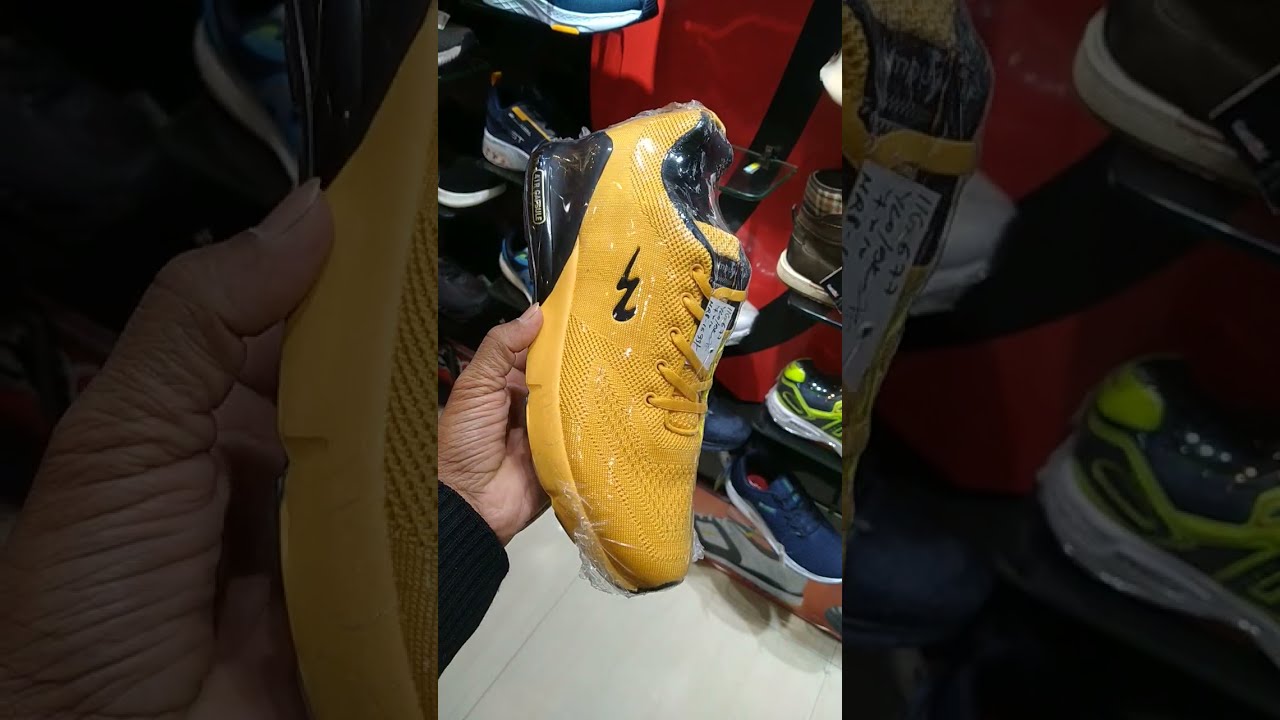The photo captures an intricately detailed scene centered around the unboxing of a distinctive sneaker. Predominantly yellow with matching laces, the athletic shoe showcases a black heel and interior lining, accentuated by a black 'W' logo. Encased in shrink wrap, the footwear is held by a man's light brown hand, emerging from the lower-left corner of the image. His blue sweater clad arm suggests this is a deliberate showcase. The background reveals a vibrant sneaker store, characterized by a red wall adorned with black stripes and numerous plastic shelves, each displaying individual shoes. The white tiled floor further accentuates the organized setting, underscoring the retail environment. Notably, the sides of the main image feature blown-up, grayed-out details, adding a layered, dimensional effect that highlights specific elements like the hand and the shoes on the shelves.